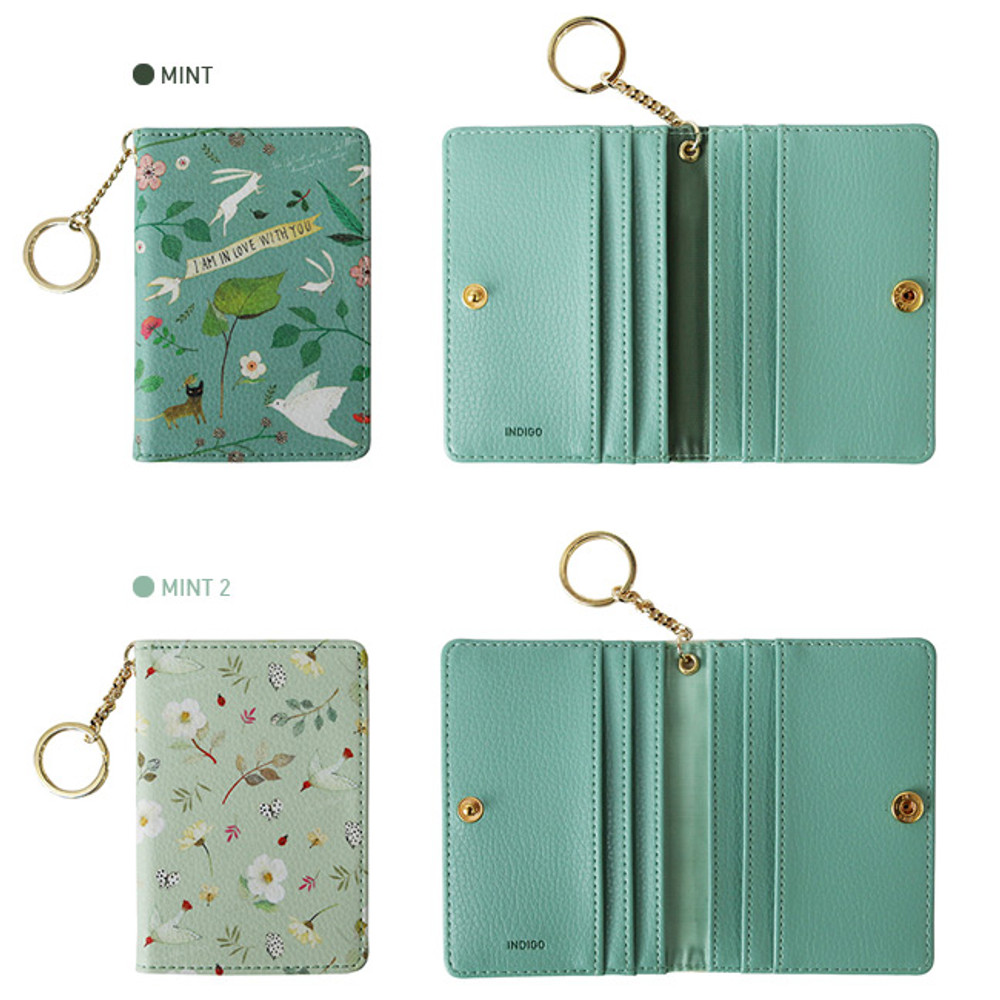The image is a detailed product display of two wallets, showing both their external and internal designs. The wallets are positioned with the darker Mint wallet at the top and the lighter Mint 2 wallet at the bottom. Both wallets are adorned with intricate designs featuring flowers, birds, butterflies, leaves, and branches in a mix of green, white, yellow, and red tones. Each wallet has a golden keychain attached to the left side and displays the text "I am in love with you" on the exterior. The insides of both wallets are a darker green and similarly structured, with sections for money and card inserts. The word "Indigo" is printed in black on the interior of each wallet. The names "Mint" and "Mint 2" are labeled near the corresponding wallets, delineating the darker and lighter green colored products respectively. This visually rich image thoroughly details the design elements, color palette, and functional aspects of the wallets.